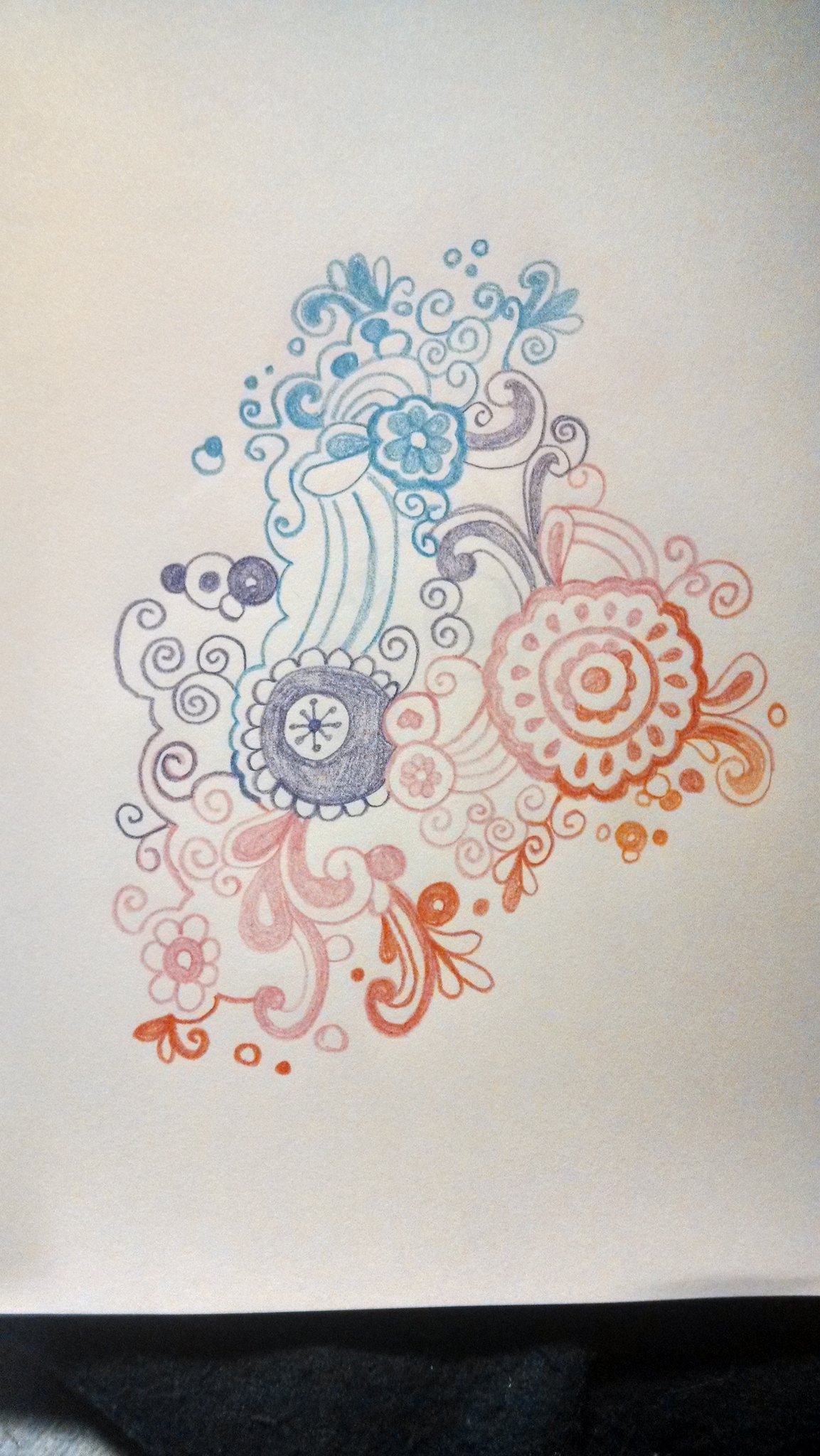Detailed Caption:

A whimsical sketch adorns a sheet of paper, bathed in soft, ambient lighting. The artwork features a dynamic composition of flowery, bubbly shapes that seamlessly flow into one another. The colors, while distinct, blend harmoniously without intermixing. At the top of the sketch, light blue hues dominate, creating a serene atmosphere. Gradually, the colors transition into subtle gray and delicate violet shades in the middle section. As the eye moves downward, the palette shifts to enchanting purples and playful pinks, finally culminating in vibrant orange tones. The sketch, though abstract and not resembling any specific object, captivates with its colorful and imaginative design.